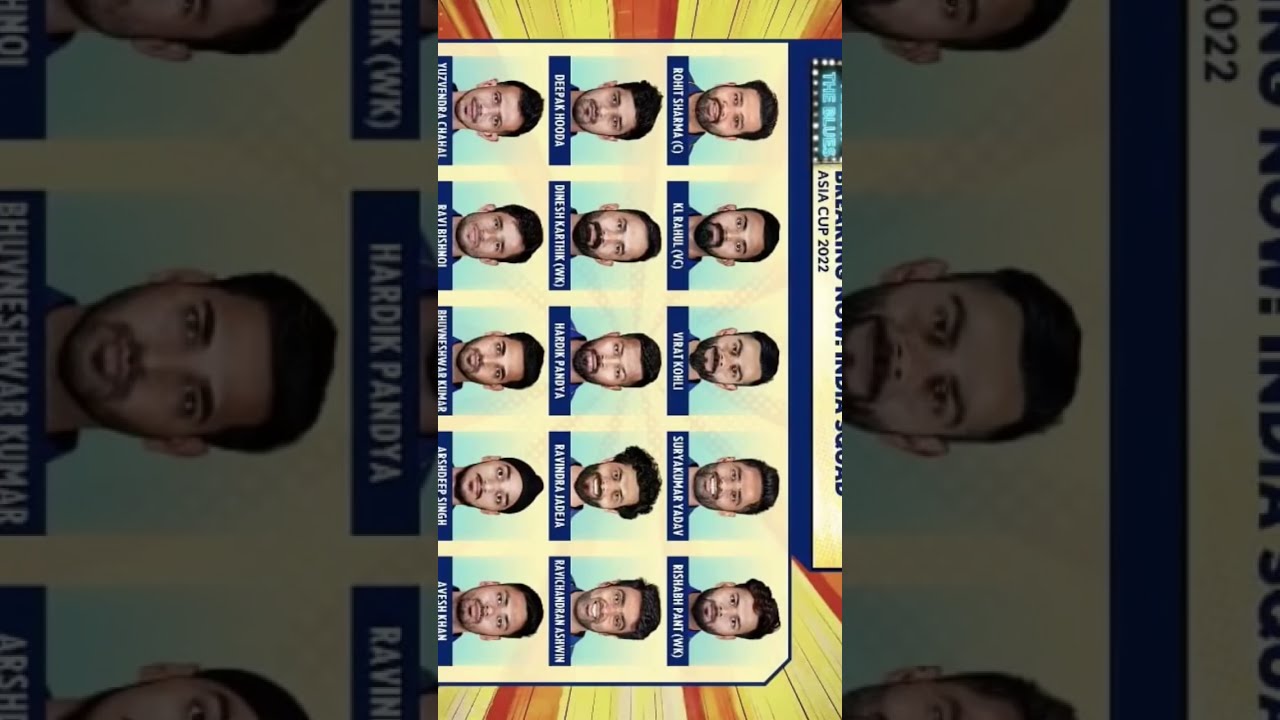The image features a series of rows of headshots depicting various men, turned sideways at a 90-degree angle. The men appear to be of East Asian descent, potentially Indian, with similar features including diverse hairstyles, facial hair such as mustaches and goatees, dark brown to black hair, and varying shades of brown skin. The headshots are well-organized, covering the entire image. Each person's name is displayed in a white font within a blue box beside their photo, though the compression makes some names hard to read. Notable names include Risaharma, Kyle Riel, Rick Coley, Samanian Yadavi, Rishavir Pant, Deepa Hukka, Dashankini, Hazuka Payoka, Revuka Aranya, and Razakira Askedaron. The top of the picture (or the right side, considering the sideways orientation) is partially cut off but clearly reads "Asia Cup 2022," suggesting these individuals could be participants in a related event. The photo appears to be a screenshot from a mobile device and showcases a color palette of yellow, red, orange, white, black, and various shades of blue.